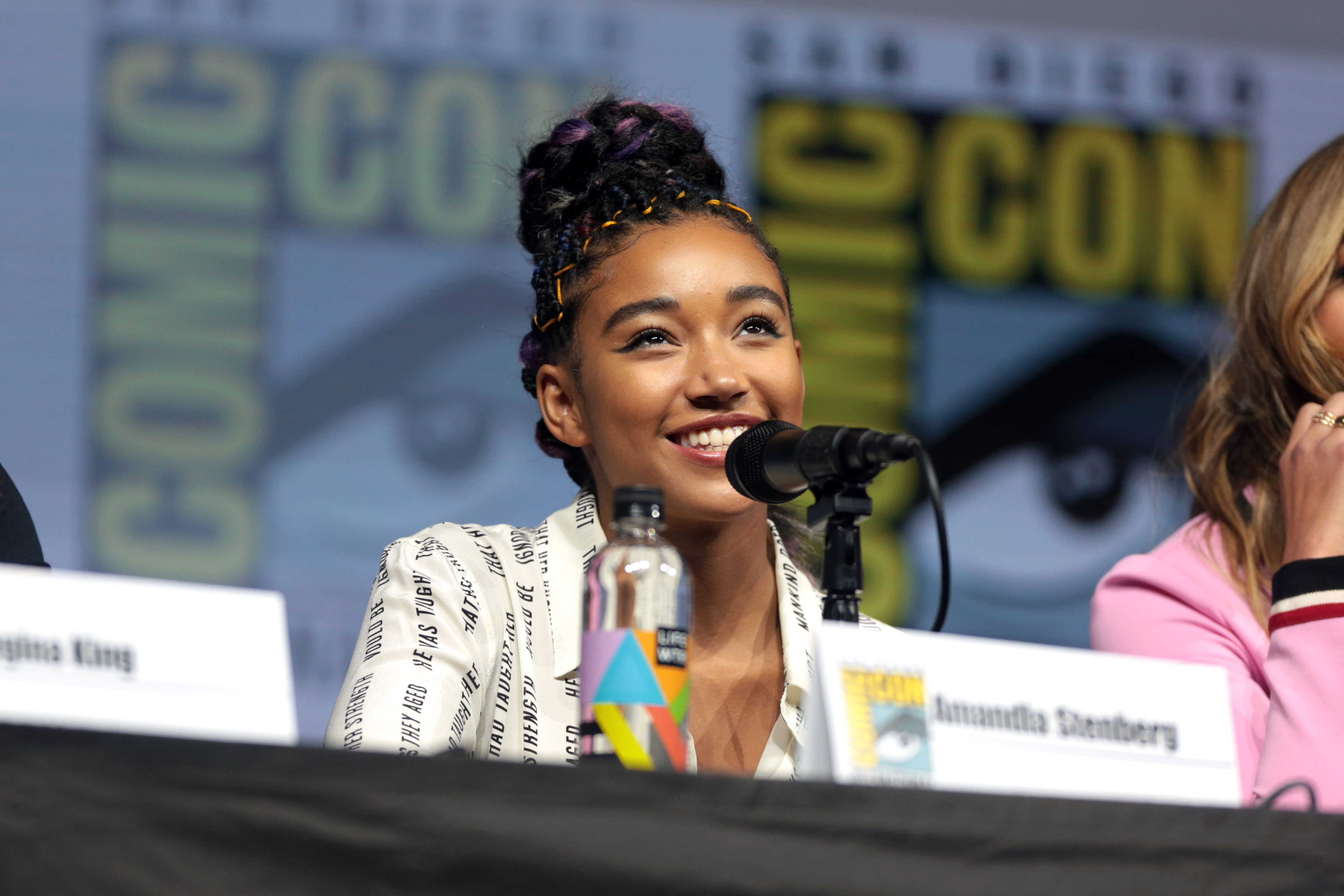This photograph captures a lively moment at San Diego Comic-Con, featuring a Hispanic woman named Amanda Stanberg. She is seated behind a table, her face radiant with a broad smile and her mouth open as she speaks animatedly into a small black desk microphone. Amanda has her black hair tied up in a large bun and is dressed in a white shirt adorned with black-font designs, though the text is obscured by the wrinkles in her clothing. In front of her lies a white name placard bearing her name, 'Amanda Stanberg.' A water bottle is also placed on the table, adding to the scene’s casual yet professional ambiance.

To Amanda's right, partially visible, is a blonde woman in a pink shirt, while to her left, another cropped figure wears black, identified only by a placard with the word 'King' on it. The backdrop behind them features a series of posters with somewhat blurred text, prominently displaying "San Diego Comic-Con" with "Comic-Con" highlighted in bold, all-caps yellow. The image conveys a warm, engaging atmosphere, with Amanda at the center, contributing to the spirited environment of the event.